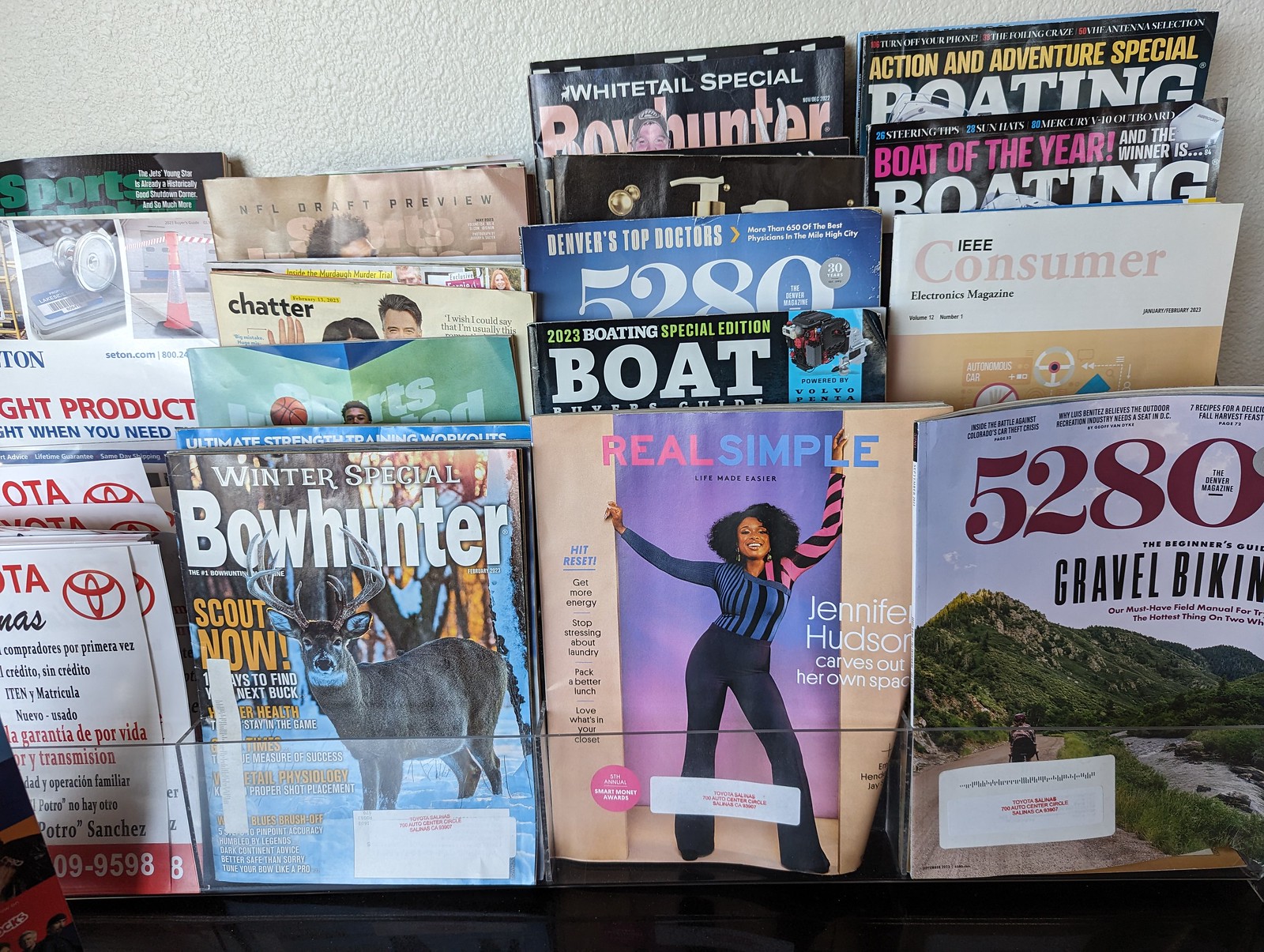The photograph showcases a rack filled with a diverse assortment of magazines neatly lined up next to each other. Among the visible titles are "Bowhunter," "Real Simple," "5280," and "Consumer." Additionally, multiple issues of "Boating" and "Bowhunter" can be seen, as well as copies of "Sports Illustrated," which include special editions like the "Winter Special Boat Hunter" and the "NFL Draft Preview." There are also some pamphlets, including one for Toyota, alongside other magazines such as the "IEEE Consumer Electronics Magazine" and "Denver's Top Doctors 5280." The covers feature various pictures and red-lettered labels, although the text on some of them is too small to read clearly.